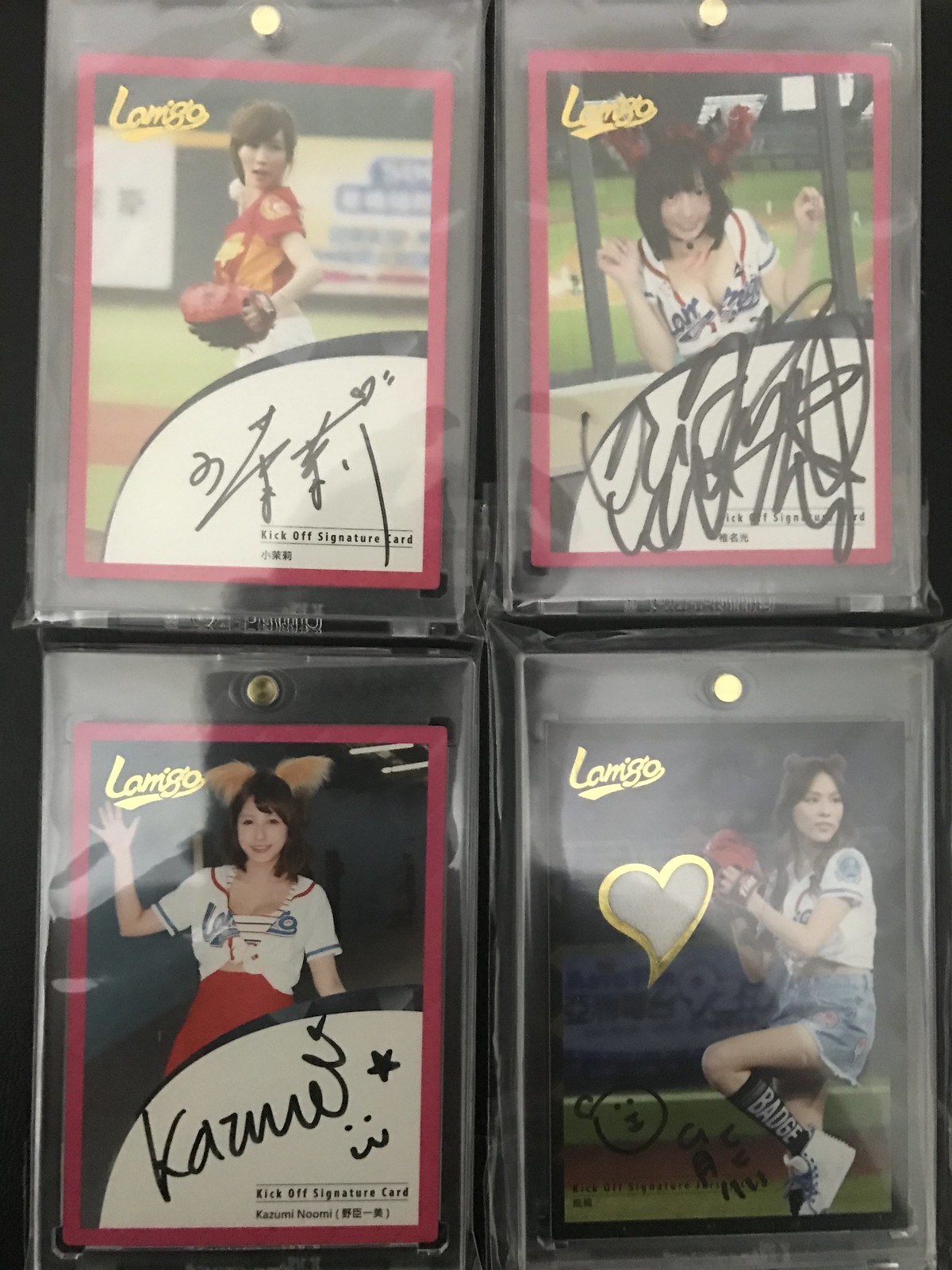The image showcases four baseball cards featuring a young Asian woman, displayed against a black wall. Each card is protected in a plastic card holder and arranged neatly. The woman is depicted in various poses: two showing her pitching in different uniforms, one where she is standing and waving, and another where she appears excited. All four cards are autographed, with three featuring a white oval area in the corner designated for the signature, while the fourth lacks this feature but still contains her autograph. The cards also contain some text and a logo in the top left corner, which reads "LONGIGO" in cursive script.